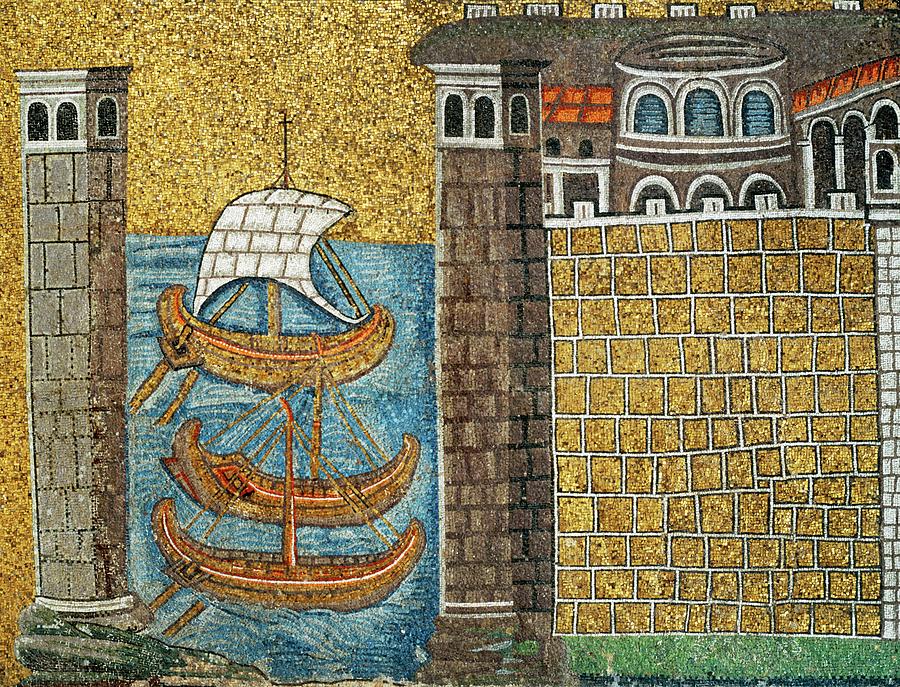The image is an intricate and detailed artistic representation of a medieval castle, reminiscent of something from a children's book. The artwork appears to be crafted with beads, giving it a distinct texture and aesthetic. The central focus is a grand, gray castle with multiple features. The castle has several blue, arched windows and is composed primarily of gray bricks. Surrounding the castle, there's a tall, gray guard tower on the left, also with arched windows; mirrored on the right by a tower with similar architectural characteristics.

Enclosing the castle is a tall, brown brick fence. To the left of the castle, there's a moat depicted in blue, housing three boats. The top boat is distinguished by a white sail, while the other two boats lack sails and have blended hues of red, gold, and brown. The overall background is a grainy mustard yellow, adding an ancient, timeless feel to the piece. This striking composition not only captures the grandeur of the castle and its defenses but also the serene nature of the water with the boats, culminating in a vivid and detailed portrayal of medieval life.